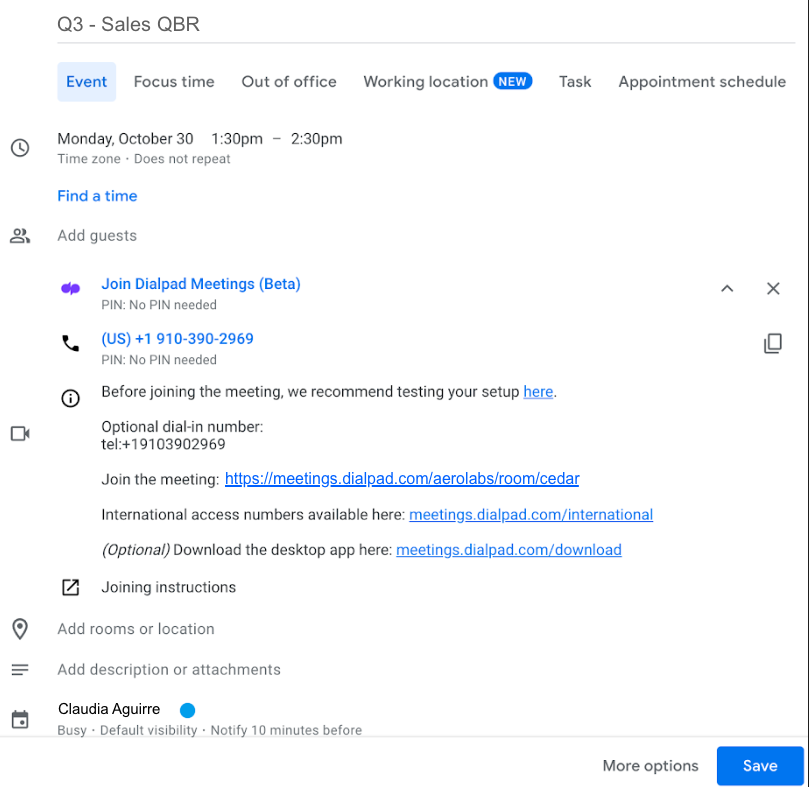This screenshot details the scheduling interface for a Q3 Sales QBR (Quarterly Business Review) event, likely within a platform such as Microsoft Teams. At the top, just below the header "Q3 Sales QBR," there are six clickable buttons providing scheduling options: Event (highlighted), Focus Time, Out of Office, Working Location, Task, and Appointment Schedule. 

The event is scheduled for Monday, October 30th, from 1:30 PM to 2:30 PM, in a non-repeating time zone. A blue clickable link labeled "Find a time" is available for easier scheduling.

Further down, there are icons for adding guests. One icon is shaded, while the other is not, indicating that guests can be added by clicking on them. 

Underneath the guest section, there are details for joining the meeting via Dialpad Meetings (in Beta). Specifically:

- PIN: No PIN needed. 
- Phone (U.S.): +1 910-390-2969.
- An optional dial-in number is +1 910-390-2969. 
- There is a clickable link suggesting to test your setup before joining the meeting.
- There are also links for international access numbers and detailed joining instructions.

Additionally, there are options to add rooms or locations, include descriptions, and specify personas for the event.